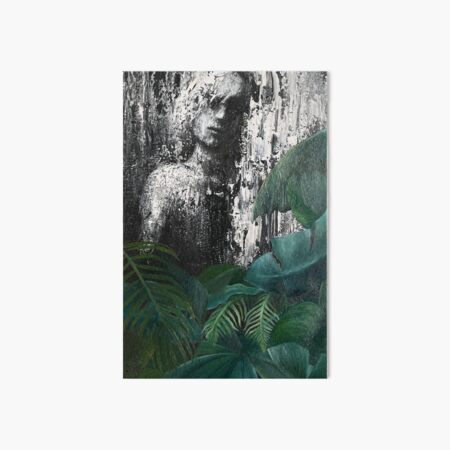This photograph showcases a portrait-style artwork, intricately blending natural elements with a human figure. The bottom half of the piece bursts with an abundant array of leaves, depicted in various shades of green, from dark and light to a faint yellow-green, even including a touch of turquoise. These leaves, predominantly large and spreading upwards, create a lush, verdant foreground that climbs partly along the sides of the artwork. The top half transitions into a monochromatic scheme of black, white, and gray, intricately forming the image of a woman. Her visage and shoulder-length hair, composed of fine lines, seem to merge seamlessly with the surrounding textures, reminiscent of tree bark or rock. The woman's form appears to emerge subtly from this background, with her face and body artfully integrated into the natural lines and contours, giving the impression of her blending into, or leaning against, the rock-like surface.